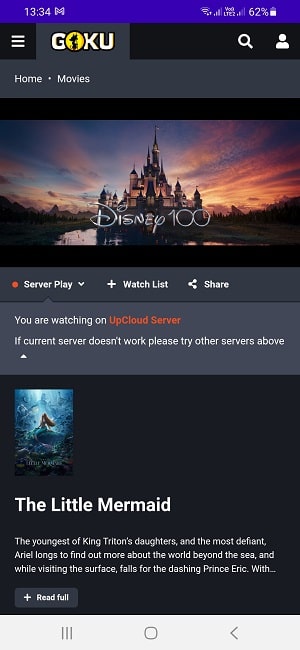The screenshot captures a moment on a smartphone at 1:34 AM, showing a battery level of 62% and an unstable signal. The screen displays a variety of content, starting with the text "Goku" followed by "Home Movies." 

Below this section lies a prominent black box, and beneath it, a vibrant image of Cinderella's Castle at Disney World, adorned with the caption "Disney 100." This iconic castle shines in all its splendor, signifying a celebration of Disney's centenary.

Further down, the screen reads, "You are watching on UpCloud server. If the current server doesn't work, please try other servers above," indicating a streaming service setup.

At the bottom of the screen, another black box contains an enchanting image of Ariel, the Little Mermaid, gracefully flicking her arm in the water. Accompanying this picture is a description: "The Little Mermaid, the youngest of King Triton's daughters and the most defiant. Ariel longs to find out more about the world beyond the sea, and while visiting the surface, falls for a dashing Prince Eric..." A clickable link or button labeled "plus full read" suggests more information is available.

The overall display provides a mixture of practical device information and enticing multimedia content, with both nostalgic Disney imagery and narrative text to engage the viewer.